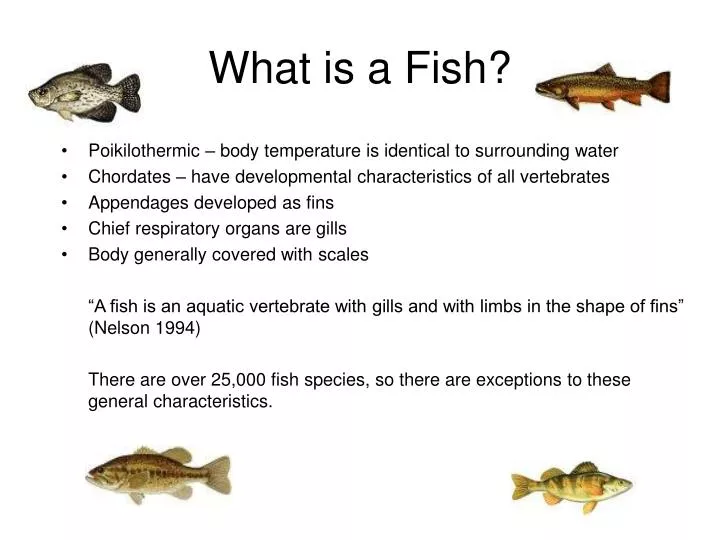This informational graphic, possibly designed for a PowerPoint slide or an educational website, features a primarily black-and-white design with a white background and black text. Each corner of the graphic includes a vibrant image of a different fish, varying in size and color: the top-left and top-right fish are facing left, while the bottom-left fish faces left and the bottom-right faces right. Notably, the top-left fish is gray, the top-right is an orangey-yellow-brown, the bottom-left fish is light brown with white, and the bottom-right fish is white with yellow.

Centered prominently in large text is the question, "What is a fish?" Below this heading, five key characteristics of fish are listed in bullet points: 
1. Pikey, low thermic – body temperature identical to surrounding water
2. Chordates – developmental characteristics of all vertebrates
3. Appendages develop as fins
4. Chief respiratory organs are gills
5. Body generally covered with scales

Additionally, there is a quote defining fish: "A fish is an aquatic vertebrate with gills and limbs in the shape of fins," attributed to Nelson, 1994. The graphic also notes that there are over 25,000 fish species, acknowledging that exceptions to these general characteristics exist. This graphic serves as a primer on the definition and basic characteristics of fish.